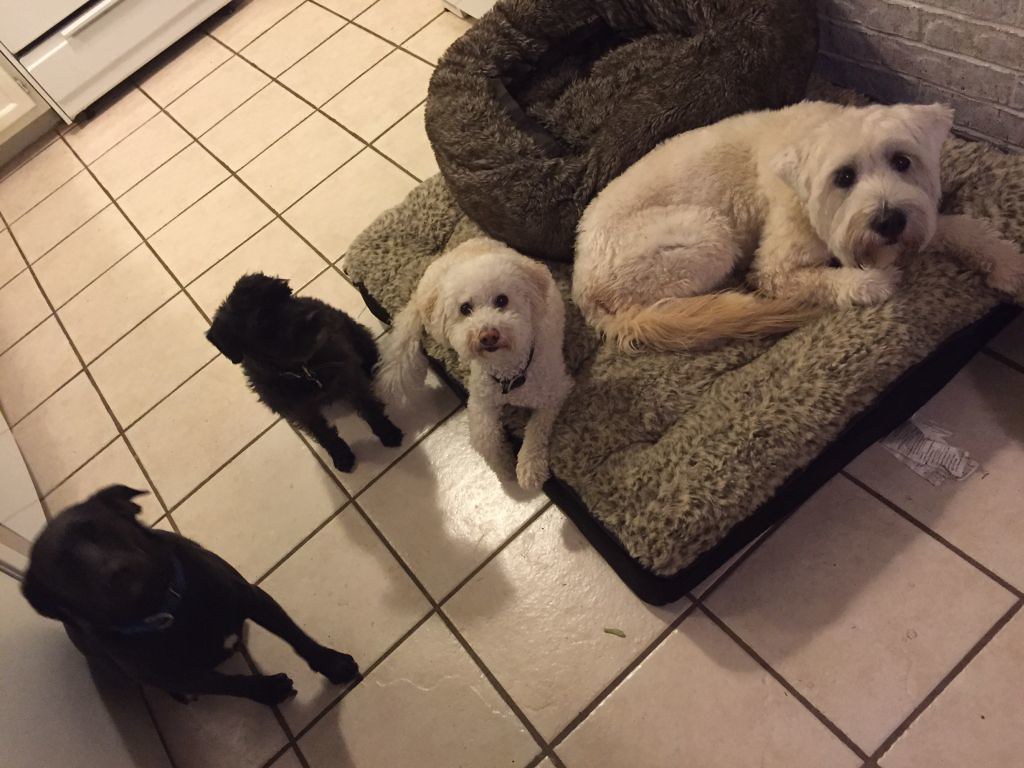This image depicts a scene with four dogs positioned on a light-colored ceramic tile floor. Two white, fluffy dogs, likely a cockapoo and a poodle mix, are settled on a large square dog bed that has a smaller round bed on top of it in the corner. The dogs on the bed appear to be adult and show mixed emotions, ranging from excitement to puzzlement. On the floor, a black Labrador with a blue collar sits up against the left wall, gazing attentively at the camera. Next to it, a small black schnauzer is seen looking off to the right. The overall setting suggests an environment where the dogs are comfortable and curious, with some displaying hints of fear.